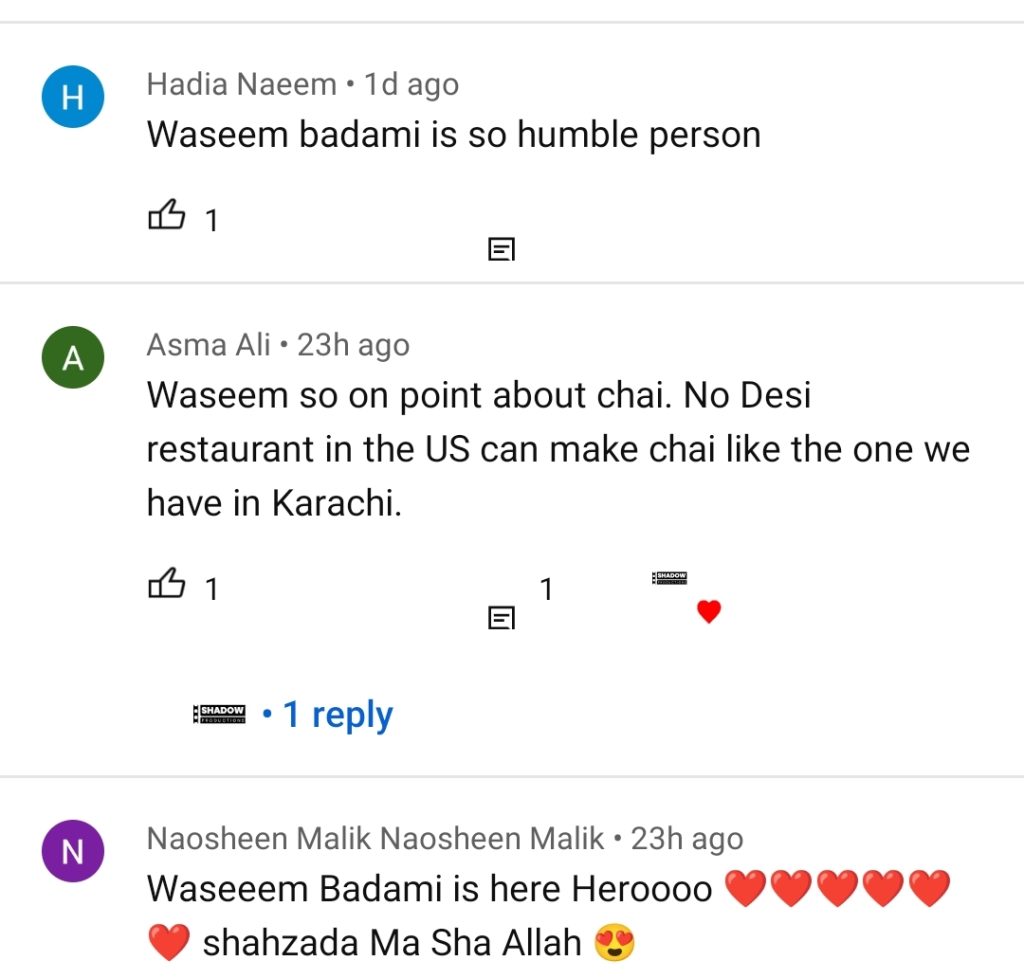The image displays three YouTube comments under a video that is not visible. The first comment, posted by Hadia Naeem one day ago, features a profile picture that is simply the letter 'H' on a blue background. Hadia wrote, "Wasim Badami is so humble person," and this comment has received one like with no replies.

The second comment is written by Asma Ali and was posted 23 hours ago. Asma's profile picture shows the letter 'A' on a green background. The comment reads, "Wasim so on point about chai; no desi restaurant in the US can make chai like the one we have in Karachi." This comment received one like, has one reply, which is not fully visible, and has been hearted by the channel creator.

The third comment comes from Naushin Malik, also posted 23 hours ago. Naushin’s profile picture is the letter 'N' against a purple background. The comment enthusiastically states, "Wasim Badami is here hero," alongside six red heart emojis, followed by the phrase "Shahzada mashallah" with a heart eyes emoji.